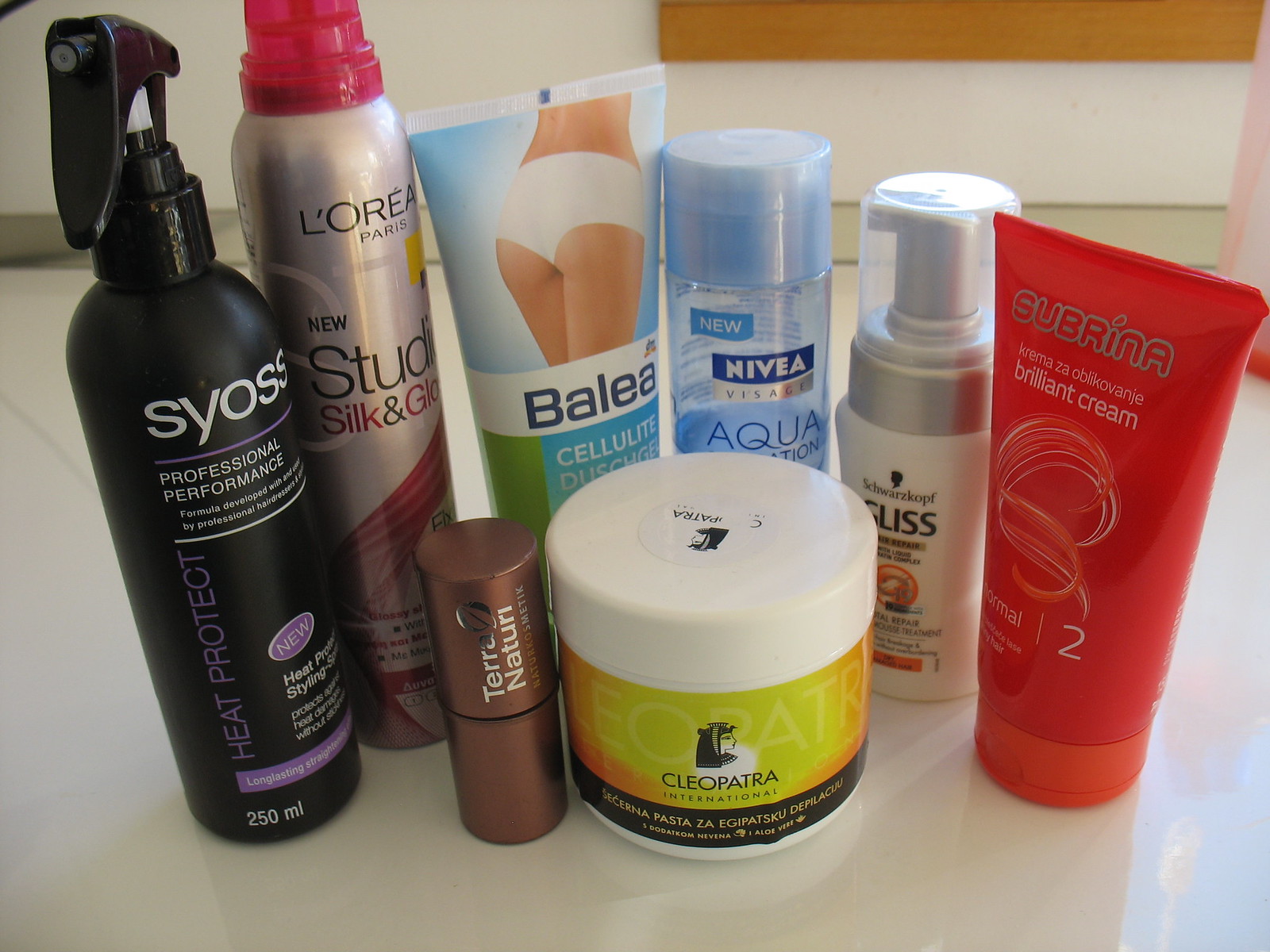This photograph showcases an orderly row of various health and beauty products displayed on a pristine white surface. From left to right:

1. A sleek black spray bottle featuring a convenient spray tip. The bottle is labeled "Syoss" in bold white font.
2. A sophisticated silver canister topped with a vibrant red cap, branded "L'Oreal New Studio Silk and Glow".
3. A plastic tube containing cellulite treatment fluid by Balea, adorned with an image of a woman's derrière clad in white panties, depicting a Caucasian complexion.
4. A robust blue plastic canister labeled "Nivea Aqua".
5. A clean white plastic canister with the brand name "Gliss" inscribed in black letters.
6. A striking red plastic tube marked "Subrina Brilliant Cream", highlighted with a graphic of curly hair.
7. In front of these products sits a white plastic tub labeled "Cleopatra" with a cheerful yellow label.
8. Adjacent to the tub, a small brown container resembling a lipstick tube completes the collection.

Each product stands distinctly, emphasizing the variety in packaging and branding within the realm of health and beauty.